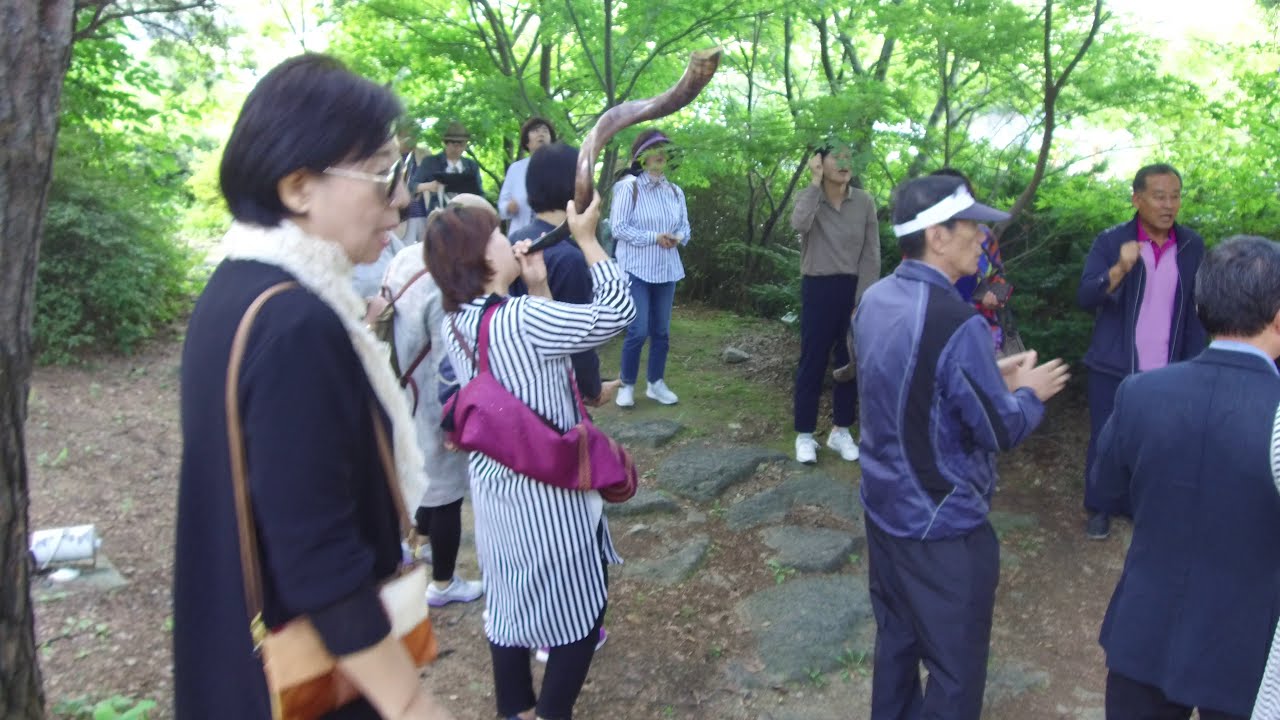In this horizontally aligned rectangular photograph taken during the daytime, a group of predominantly Asian individuals is gathered in a wooded park area with a dirt and rocky ground. Green leaves and tree trunks frame the background, with sunlight filtering through. The group, a mix of males and females, including some elderly, is casually dressed in jeans, sneakers, and various blue and dark-colored jackets with a few wearing caps and visors. One standout woman with short black hair and a blue jacket with white fur around the collar is holding a purse. Another woman in the center, dressed in a vertically striped black and white long shirt over black pants, is playing a wooden flute reminiscent of a traditional Mongolian instrument, suggesting a celebratory or ceremonial event. She draws attention as the focal point, while a man in a purple shirt appears to be cheering. Everyone faces towards the right, where the scene cuts off, leaving an air of curiosity about what might be happening off-frame.